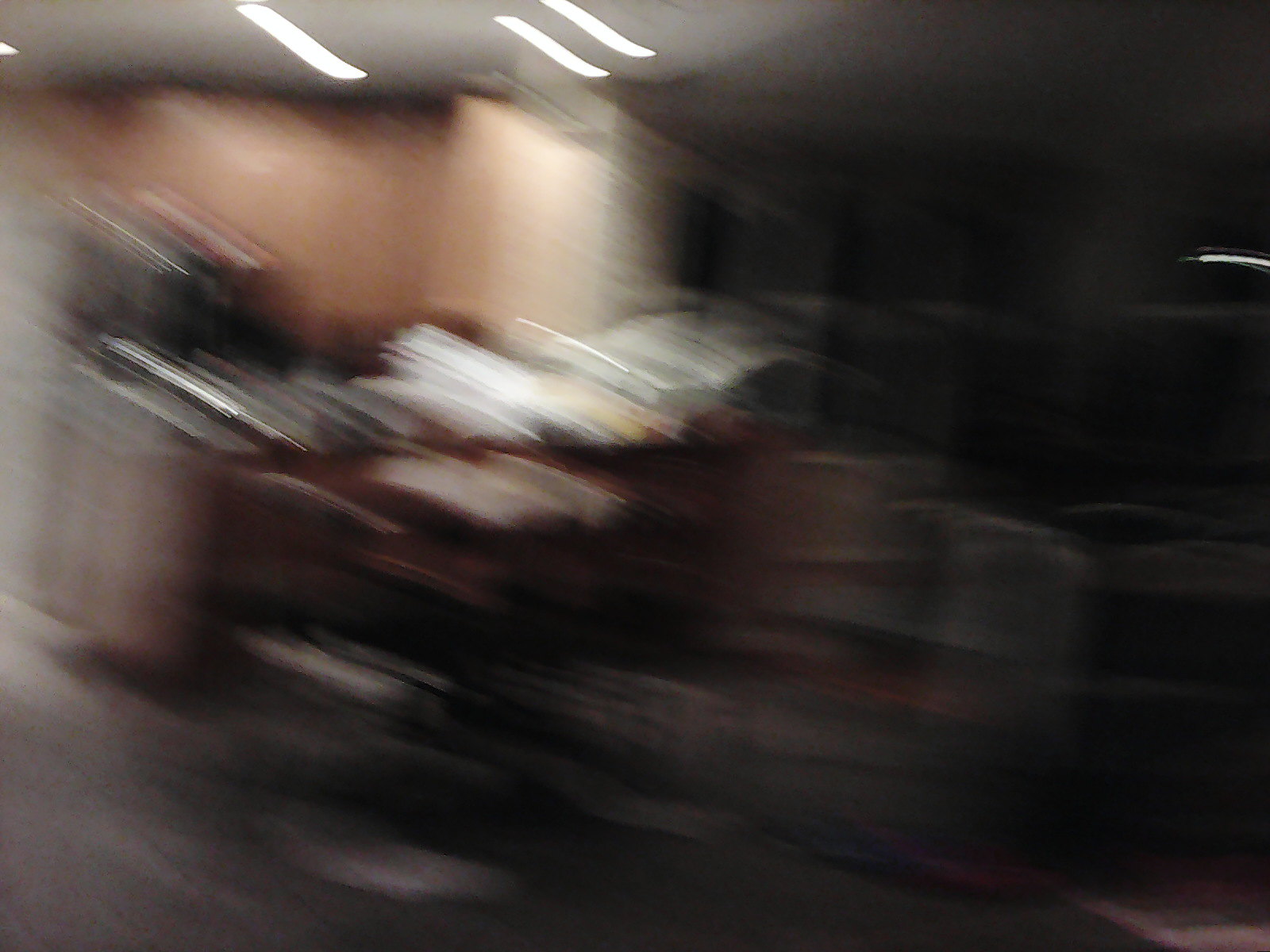The photograph is highly blurry, capturing what seems to be a room. The image includes bright white lights at the top, possibly from office ceiling lights or spotlights. The right side of the photograph is very dark, obscuring details, while the left side is brighter and slightly overexposed. The picture appears to have been taken in motion, creating diagonal or radial blur patterns that make distinguishing specific shapes difficult. The bottom of the photo transitions into different shades of gray and black with hints of white. Overall, the photograph resembles an abstract painting due to its indiscernible, smeared quality.